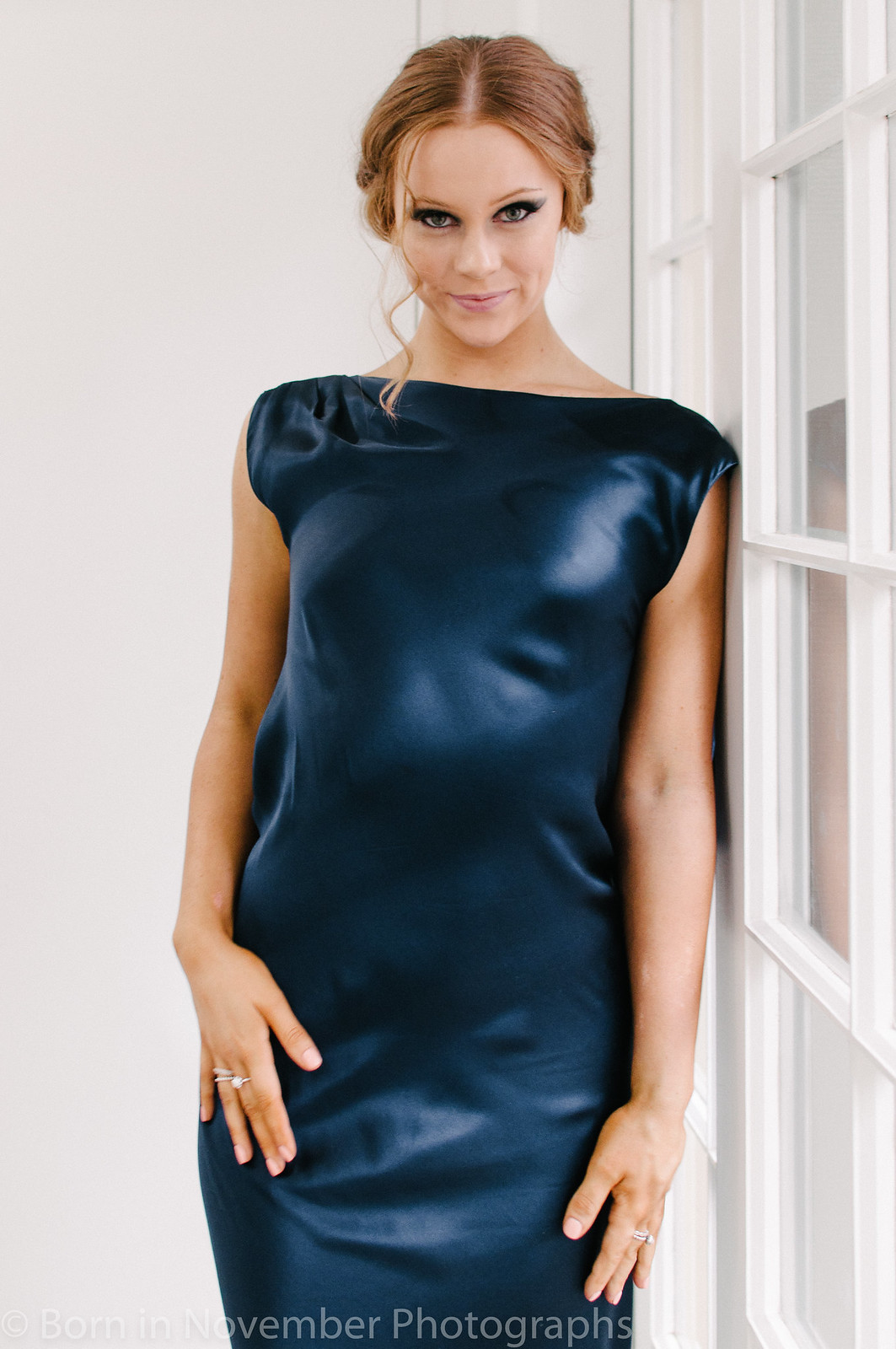The image features a woman with reddish-brown hair pulled up and behind her head, standing against a white background that includes a door with window panes. She has blue eyes and a smile on her face. The woman is dressed in a dark navy blue, off-the-shoulder evening gown that shimmers and falls between below the knee and above the ankle. Her hands are resting on her legs, and she is adorned with multiple rings: one on her right middle finger, two on her right ring finger, and one on her left middle finger. At the bottom of the image, white text reads "Born in November Photography."